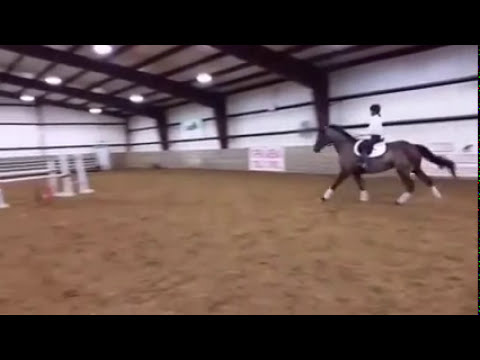A blurred photograph captures a rider on a black horse in an indoor equestrian training area. Both the horse and rider are moving to the left, with the horse's left legs extended forward and its back right leg arched. The horse has a black tail and is equipped with white wrappings around its legs, while the rider, whose face is indiscernible, has black hair and wears a white shirt, black pants, and possibly a black helmet. The horse is saddled with a white saddle. The training area features a dirt ground, obstacles possibly used for jumping on the left, and a white enclosure with brown and black beams. The facility's interior has wooden beams supporting the ceiling, which also holds lights. The rectangular image is framed with black borders on the top and bottom.